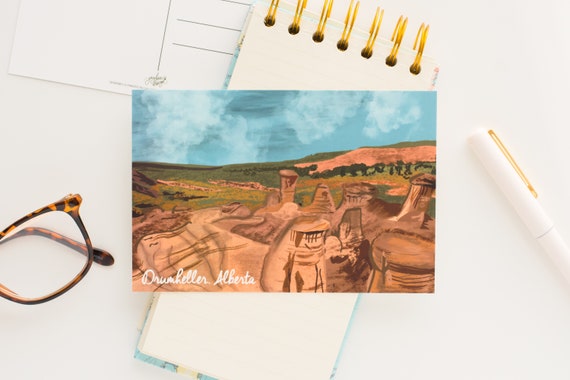This image displays an overhead view of a clean white desk. At the center sits a prominent postcard with the words "Drumheller, Alberta." The postcard features an illustrated scene showing a blue sky with clouds, grassy-topped and rocky beige mountains, suggesting a desert-like landscape, complemented by a possible design element or statue atop one of the mountains. Underneath the postcard lies a small spiral notepad with gold metal spirals, and behind this notepad is the reverse side of the postcard, showing its blank address and message sections. To the left of the postcard is a pair of tortoise shell glasses, partially visible and folded. On the far right side of the image rests a white pen with a gold clip, adding a touch of elegance to the setting. The overall composition has a balanced, organized feel and subtly suggests that the objects are computer-generated.